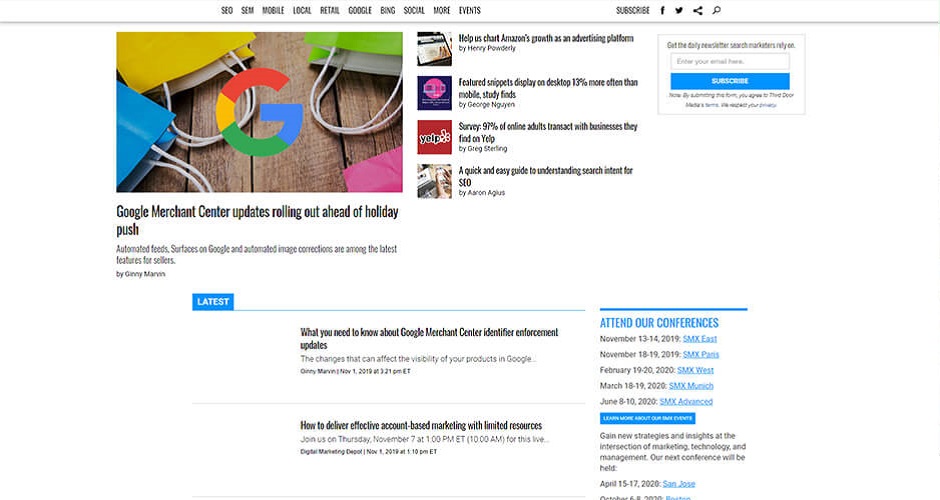This image is a screenshot of a technology news website. At the very top, the website features navigational tabs labeled "Mobile," "Local," "Retail," "Google," "Bing," "Social," and others, providing easy access to different categories of tech news. To the right of these tabs, there's a “Subscribe” button, allowing users to subscribe to the website. Additionally, there are shortcuts to the website’s social media pages on Facebook and Twitter.

Below this navigation section, a significant part of the screen displays various news listings and posts. The prominently featured article, which takes up most of the screen, is about Google. The headline reads, "Google Merchant Center Updates Rolling Out Ahead of Holiday Push," accompanied by an image of a wooden table with a large Google logo in the center. 

To the right of the featured post, there are smaller-font posts further detailing other news items. Below these, there is a “Latest” section showing a chronological listing of news posts, indicating the most recent updates and developments in the tech world.